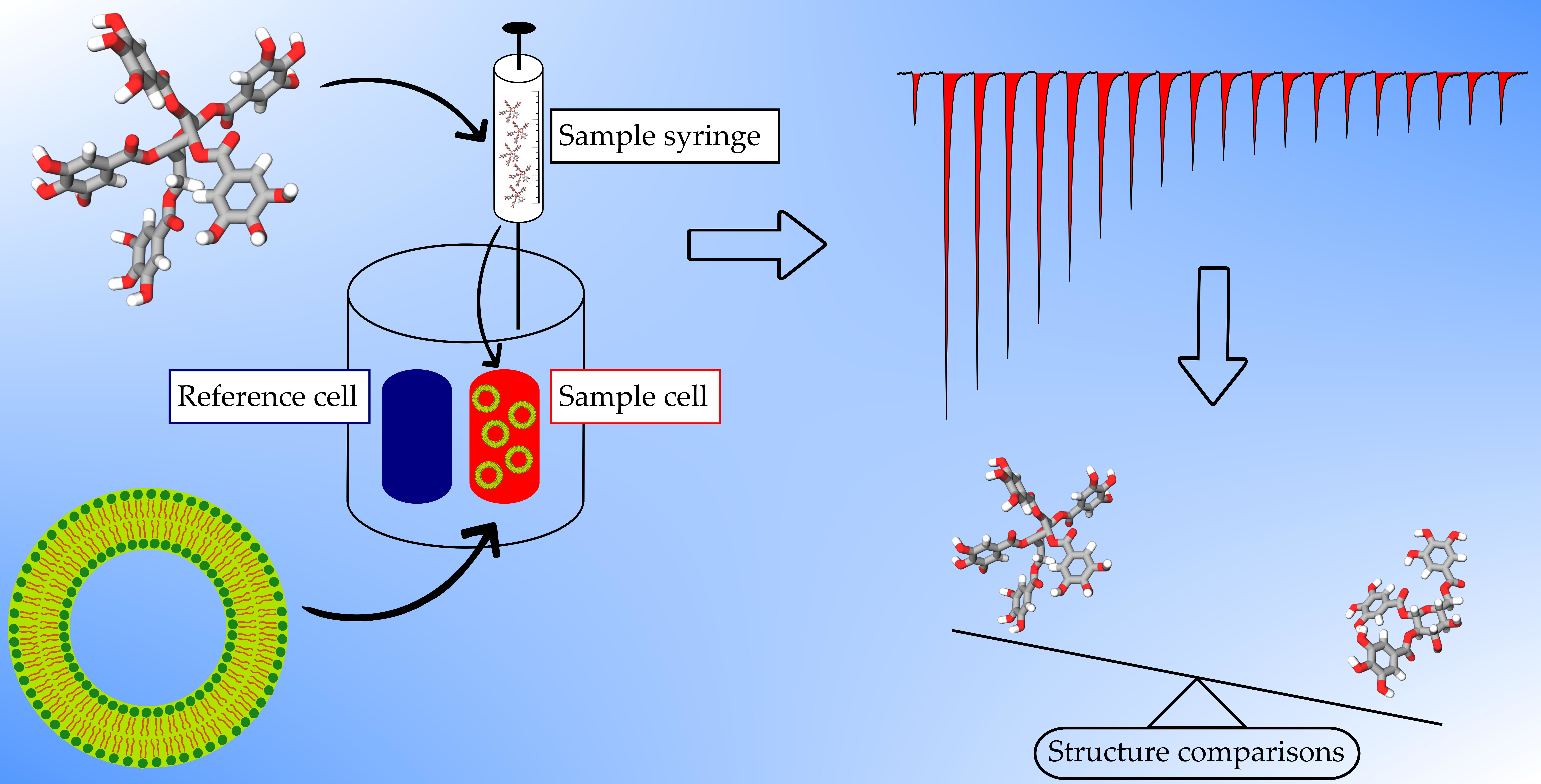The image depicts a detailed biochemical testing process on a blue, sky-colored background with various light blue highlights. In the upper left corner, there is a complex molecule composed of red, white, and gray hexagonal shapes, representative of a polyol with five sugars attached via ester linkages. An arrow points from this molecule to a sample syringe filled with miniature versions of the molecule. The syringe is shown injecting into a transparent outer cylinder containing two inner cylinders: a blue reference cell and a red sample cell, the latter adorned with yellow rings that represent a lipid bilayer, potentially indicating liposomes or vesicles.

On the upper right side of the image, there is what appears to be a chromatogram with red peaks of varying heights. These peaks start low, build to a prominent apex, and gradually decline back to the initial height. Below this, there's an iconic structure comparison involving a seesaw-like balance. One side of the balance holds the original molecule with five sugars, while the other side holds a simplified version with only three sugars. The balance tips towards the smaller molecule, suggesting a significant difference in weight.

Overall, the meticulous details, from the molecular structure and injection apparatus to the chromatogram and structure comparison, intricately illustrate the biochemical testing process being depicted.